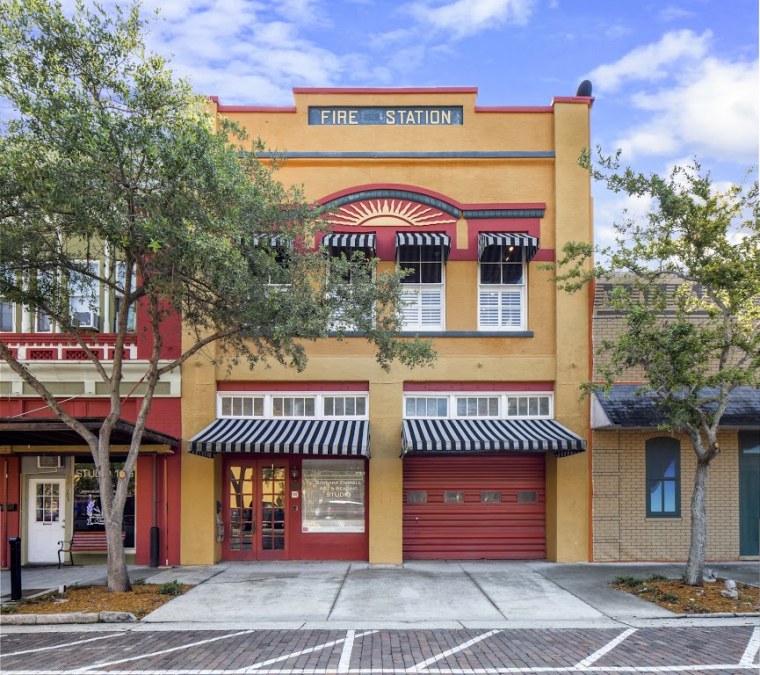The photo captures a vibrant two-story fire station seamlessly integrated into a quaint Main Street setting. The building, painted a bright orange with black framing and red accents, exudes a cheerful and lively appearance under a clear blue sky with scattered clouds. Each window and the black garage door are adorned with striking black and white striped awnings, adding a playful touch. A large, yellow sun emblem is prominently featured above the second-floor windows, which hints at a sunny locale, possibly in Arizona or California.

The fire station sign stands out with a teal green background, marking its identity clearly. The street in front of the station features neatly planted trees in dirt squares along a clean brick-paved sidewalk, enhancing the orderly and well-maintained ambiance. Storefronts on either side of the fire station are painted in harmonious hues of yellows and reds, maintaining a uniform yet colorful aesthetic. Despite its possible historical roots, indicated by the glass-paneled door with squarish glass panels and preserved architecture, the fire station appears meticulously maintained, contributing to the charming and peaceful atmosphere of this small town or city street scene.